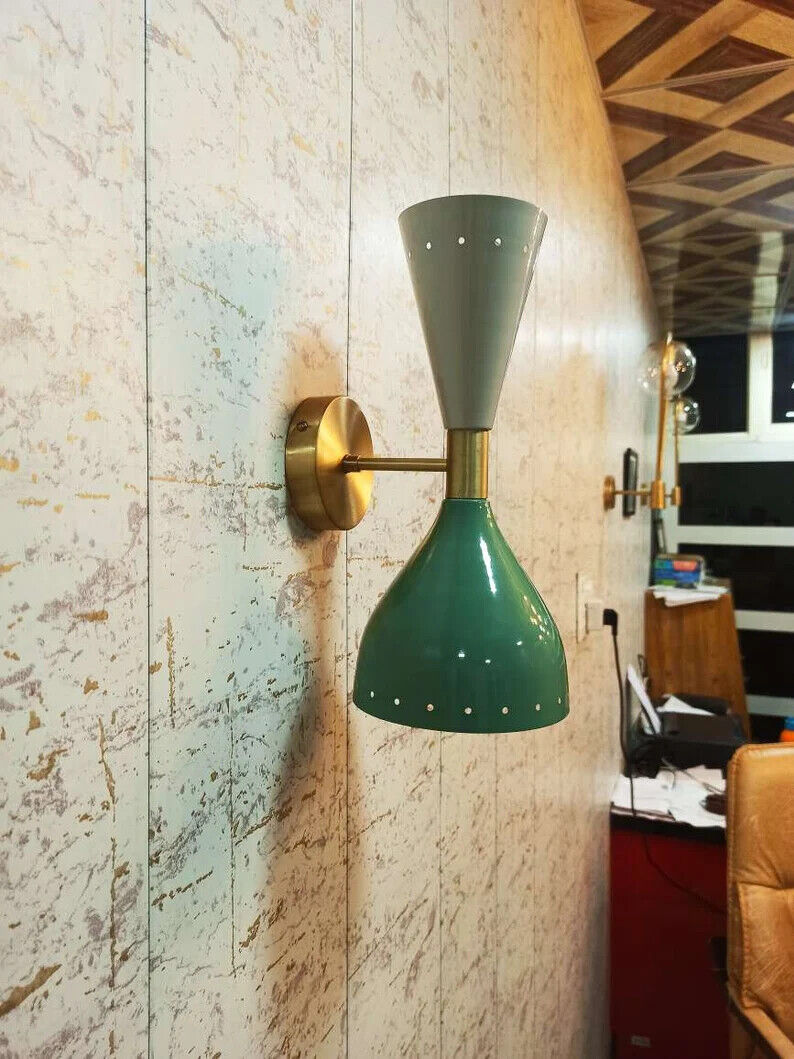The image showcases a section of a wall that appears to be covered in a tile-like or marble surface with a mix of white, gray, and brown hues, giving it a scratched, mineral-like texture. Mounted on this wall is a distinctive green light fixture with two cone-shaped lamps on either end of an extending metal pole that has a bronze base. The fixture has one larger opening at the bottom and a smaller one at the top, although it seems that light is coming only from the top. To the right of this light fixture, there is a wooden desk with a plug inserted into a socket. Above the desk, a piece of art or a clock is also affixed to the wall. Further to the right, mid-way up the wall, shelves can be seen, and at the bottom right corner, the edge of a leather chair is visible.